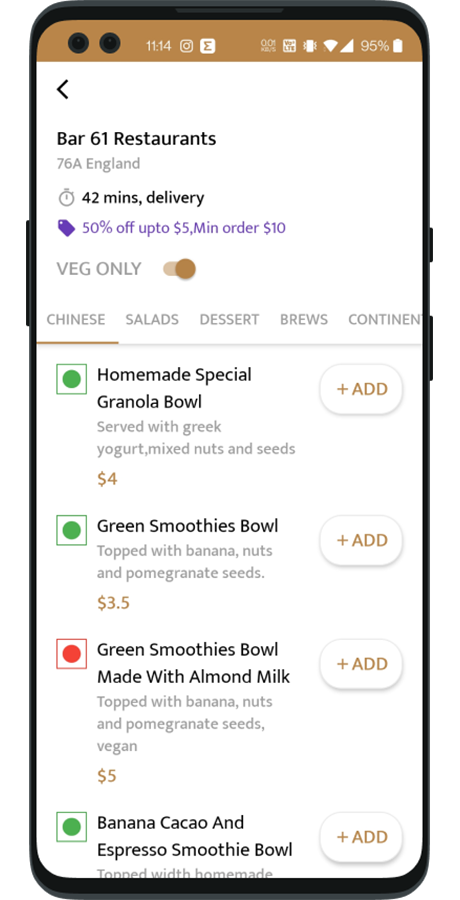Screenshot of a restaurant delivery app interface showing available vegetarian options from "Bar 61 Restaurants." The top of the screenshot features a brown bar with two camera icons. Below it, a section highlights promotional details: "42 minutes for delivery" and "50% off," with the latter written in eye-catching purple text. The vegetarian filter is enabled, highlighting the exclusively vegetarian offerings. The categories displayed include Chinese, salads, desserts, and brews.

Specific menu items are listed with their prices: 
- **Homemade Granola Bowl with Yogurt** - $4
- **Green Smoothie Bowl** - $3
- **Red Smoothie** - $5
- **Banana Cocoa** - price not specified

Some items have green squares with green circles inside, while one item has a red square with a red circle inside, indicating a special status or note. No items have been added to the cart yet.